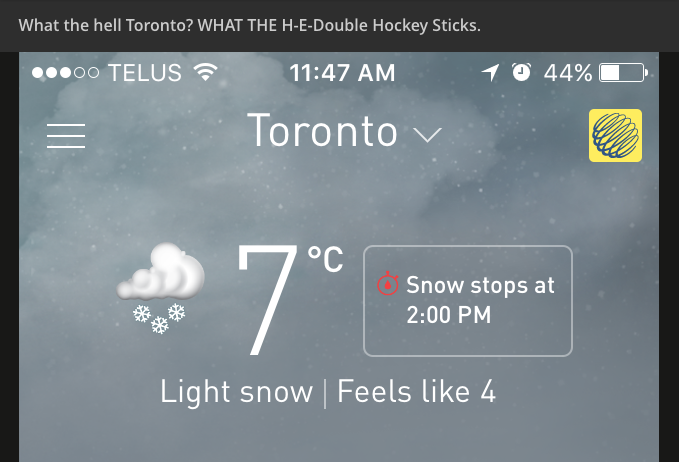The image features a weather report with a black background. At the very top, bold text reads, “What the hell, Toronto?” followed by the phrase “What the H-E double hockey sticks” in all caps. 

Beneath this heading is a screen capture of a smartphone display, showing the time as 11:47 a.m. and the battery at 44%. The location is listed as Toronto, with a weather icon depicting a cloud and several snowflakes, indicating snowfall. The temperature is displayed as 7 degrees Celsius. Next to the temperature, a white rectangle provides additional information: “Snow stops at 2 p.m.” with a small red stopwatch icon.

Further down, the screen details the current weather condition as “light snow,” stating it “feels like 4” degrees Celsius.